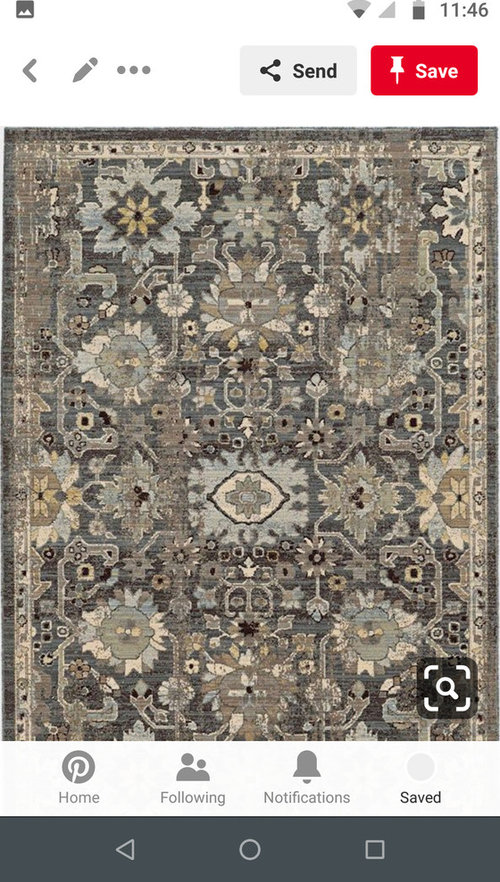The image appears to be a screenshot from a mobile device, likely an Android or iPhone, displaying an app interface in portrait mode. 

At the top left corner of the screen, there's a large white area. Within this area is a black square icon at the lower section containing white shapes that resemble mountains. On the far right of this white area, the standard Wi-Fi icon shows a weak signal indicated by completely gray bars. Next to it is a battery icon that's three-fourths full, and the current time displayed is 11:46.

Below the black square icon on the left, there is a sideways, leftward-facing gray 'V' symbol situated next to a gray pencil icon and three horizontally aligned gray dots in a row. To the right in the same row is a gray box featuring three black dots connected by lines, accompanied by the text "Send" in black letters. Following this is a red box containing a white pushpin icon labeled "Save" in white text.

Dominating the central portion of the screen is an image of a luxurious, possibly antique, Turkish or Oriental rug. This rug is decorated with intricate, almost floral, designs and various diamond patterns. The colors are primarily shades of gray and black, with accents of orange, giving the rug a vintage appearance. In the lower right corner of this rug image is a transparent black square, with white lines marking each corner and a white magnifying glass in the center, suggesting a zoom-in feature.

Below the rug image is a white area with a set of four icons lined up horizontally. From left to right: 
1. Several concentric gray and white circles labeled "Home" in gray letters.
2. An icon of two people with "Following" written below it.
3. A gray bell icon with "Notifications" in gray letters underneath.
4. A faint gray circle with "Saved" in black letters below it.

At the very bottom of the image is a long, dark gray bar containing three symbols: 
1. A play triangle filled in with gray on the left.
2. A gray-filled white circle in the center.
3. A gray-filled white square on the right. 

The entire layout suggests that the user interface portrays detailed icons and images typically found in a mobile application.